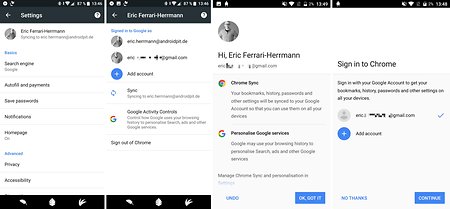Eric Ferrari Herman's Android phone screen displays the Google Chrome settings interface, indicating he is attempting to sign into his Google account. The image reveals several settings options including "Search Engine," "Autofill and Payments," "Save Passwords," "Notifications," "Homepage," "Privacy," and "Accessibility." Eric has two Google accounts on his device with the ability to add another, sync data with other devices, manage Google Activity controls, and sign out of Chrome. He is currently signed into one account, represented by an email handle ending in "@gmail." The status bar shows it is around 13:00 (1 PM) based on military time, and the device is connected to Wi-Fi. The phone has black borders, and the Google Chrome app appears navy blue on the screen. The interface provides options to continue, confirm with "OK," or undo actions.